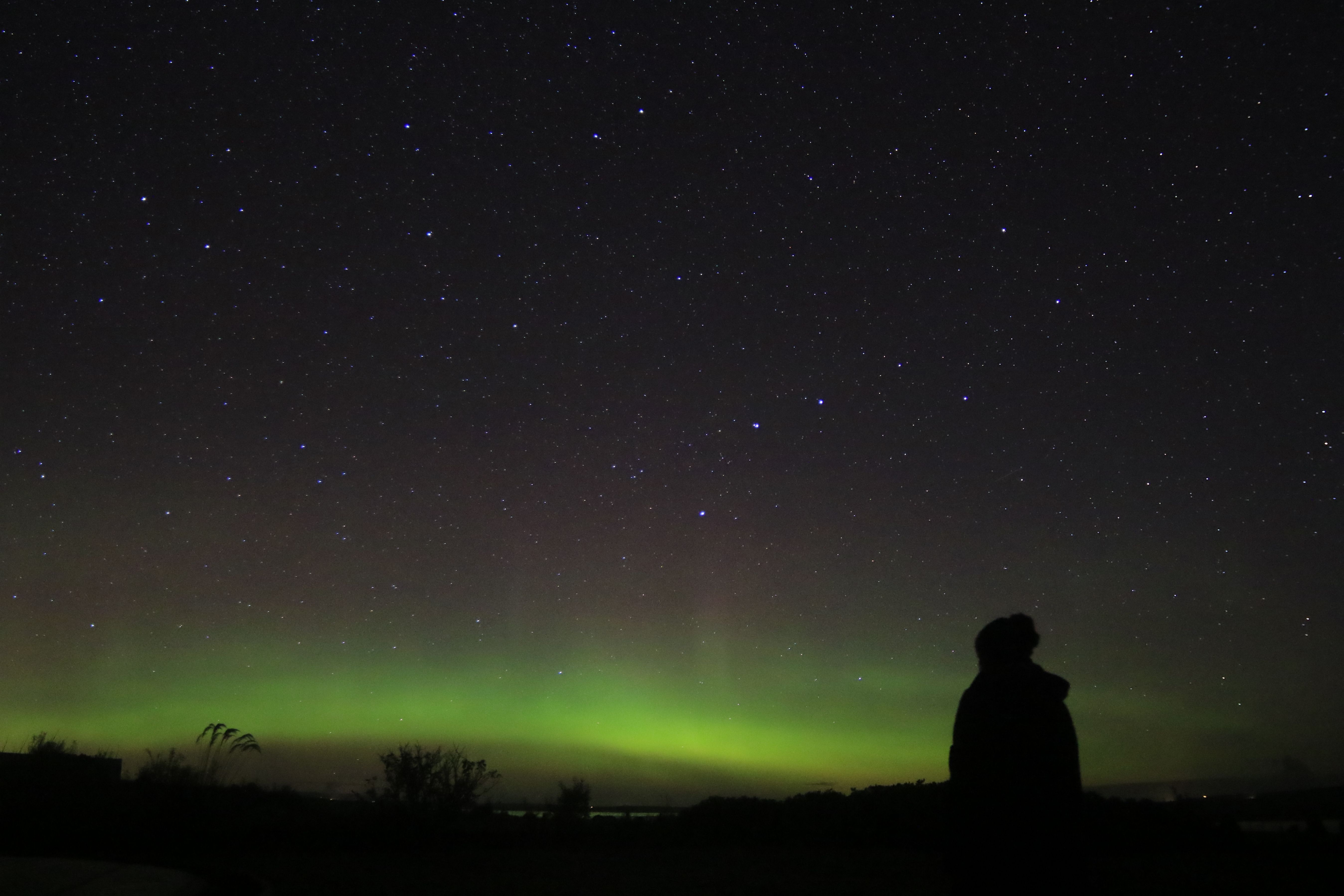This image captures a serene night sky, predominantly dark, stretching across more than three-quarters of the frame. Scattered throughout the sky are numerous twinkling stars, ranging from tiny specks to slightly larger dots. Towards the bottom third of the picture, the ethereal glow of the aurora borealis casts a vibrant neon green hue, illuminating the horizon. Silhouetted against this luminous backdrop are trees and bushes, adding depth to the scene. On a small hill, slightly to the center right, is the shadowy figure of a person. Only visible from the waist up, this indistinct silhouette gazes contemplatively at the majestic Northern Lights, their features obscured, making it impossible to determine whether they are male or female. The tranquil beauty of this scene underscores the quiet awe inspired by nature's nocturnal display.